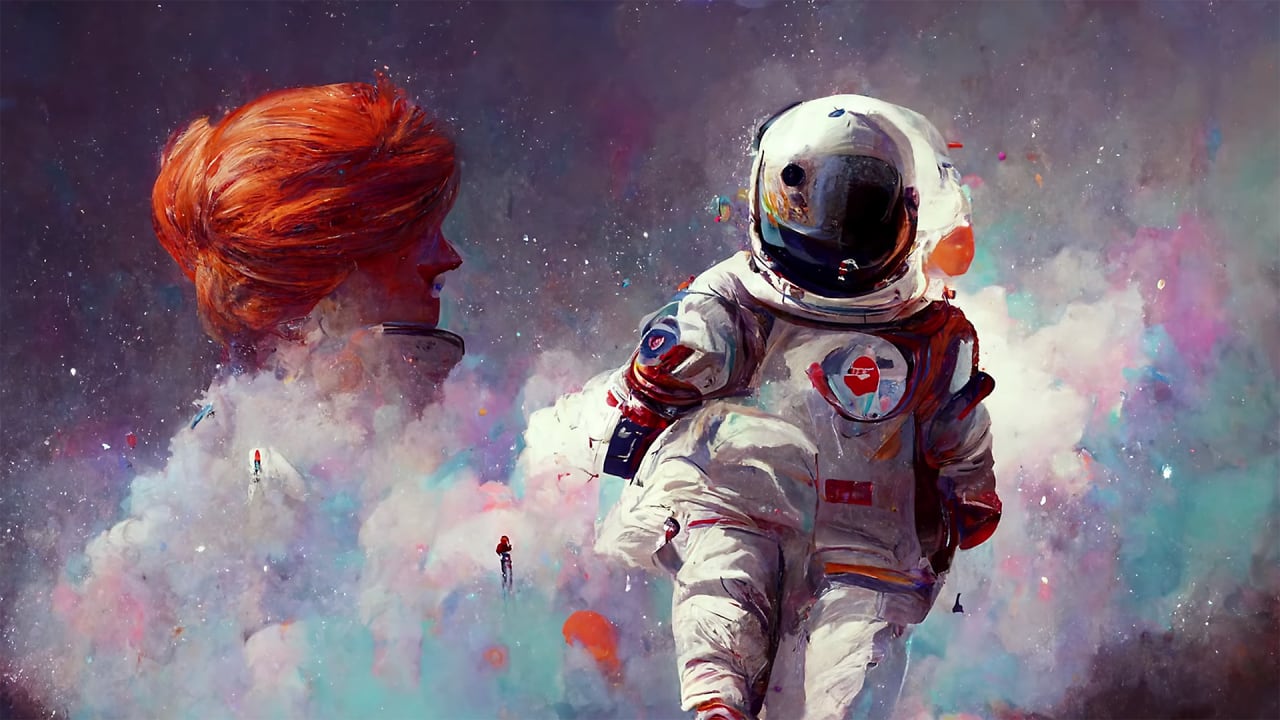This vibrant, hand-drawn or painted image, likely from the 1970s, is a colorful abstract illustration featuring a prominent astronaut and a woman with red hair. The elongated piece showcases a richly hued sky with clouds in various shades of pink, green, and white, and scattered tiny figurines floating within them. At the right center, an astronaut in a fully shaded space suit and helmet appears to be kneeling, devoid of visible arms or a discernable face. To the left, only the side profile of a woman's head with red hair pulled back in a bun emerges from the colorful clouds, creating a surreal and mystifying scene. The background is punctuated with stars, adding a cosmic touch to this complex artistic expression.